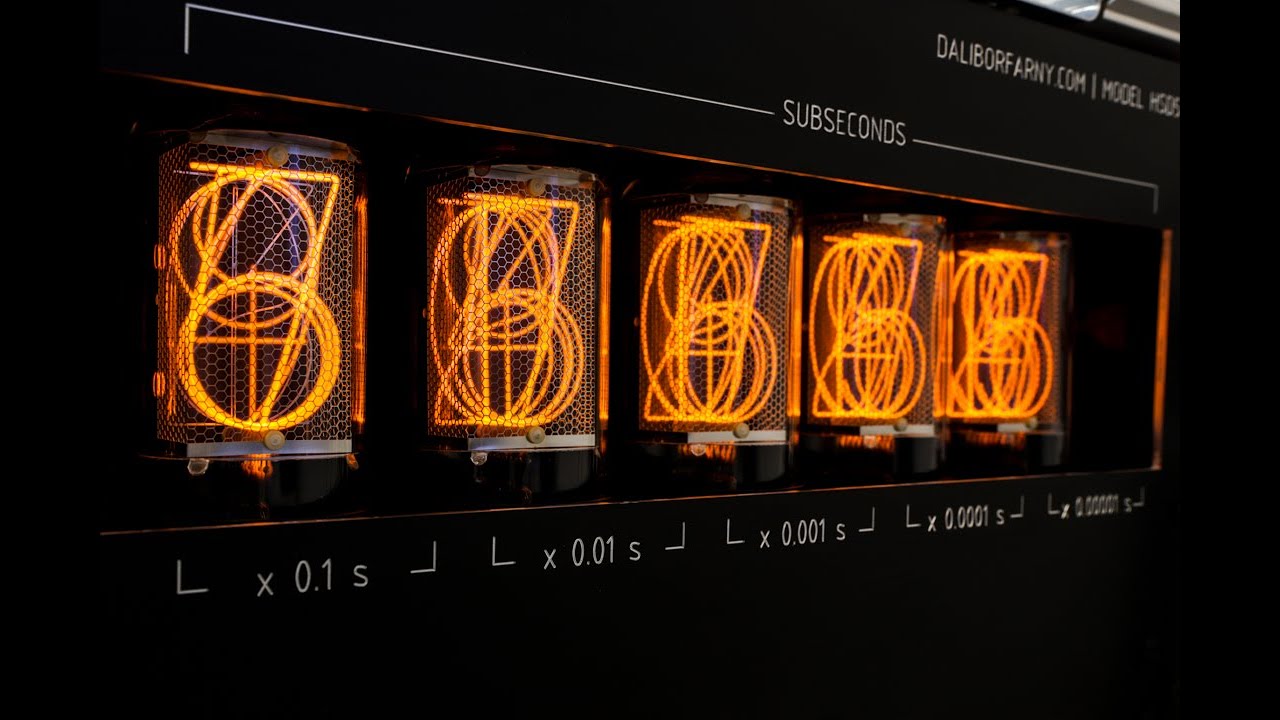The image features a very dark, almost black background, suggesting it's an electronic screen or display of some sort. In the upper right corner, white text reads "dalborfarny.com model," though the specific model number is largely unreadable and out of focus. Diagonally across the center is a line with the word "subseconds." Below this line, there are five wire-cage-like structures illuminated with overlapping, glowing orange neon numbers or electric coils, making it difficult to discern any specific numeral clearly. Each of these structures is labeled in sequence with what appears to be timing intervals, starting with "X0.1S," followed by "X0.01S," "X0.001S," "X0.0001S," and finally, an unreadable out-of-focus label. The intricate design and unusual appearance of the neon-lit structures add to the enigmatic nature of the image.